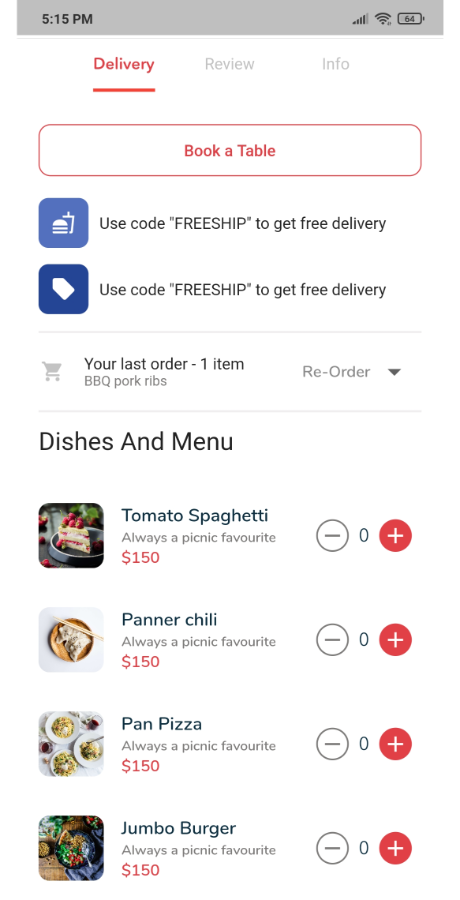At the top of the image is a long gray rectangle displaying the time on the left at 5:15 p.m., and a battery symbol on the right. Below this is a navigation bar with the word "Delivery" in red and underlined, followed by the words "Review" in light gray, and "Info." To the far right, inside a long rectangle outlined in red, the text "Book a Table" can be seen.

Beneath the navigation bar, there is a blue square with an icon and the message "USE CODE FREESHIP" in all capital letters, within quotation marks, explaining that the code provides free delivery. Another blue square accompanies this, depicting a tag icon and reiterating the same promotional offer for free delivery using the code "FREESHIP."

The image details the user's last order, stating "Your last order, one item: BBQ Pork Ribs" and provides the option to reorder.

Further down, in black text, are the headers "Dishes" and "Menu," showcasing various food items with their prices:
- "Tomato Spaghetti" ($150) depicted with an image of pasta topped with tomatoes, along with a red circle containing a plus sign to add the item.
- "Paneer Chili," described as "always a picnic favorite," priced at $150, with an option to add it.
- "Pan Pizza" displayed on white plates, available for $150 in red text.
- "Jumbo Burger," priced at $150, is shown alongside an image of a burger in a square on the left.

Each listed food item includes an option to add it to the order.